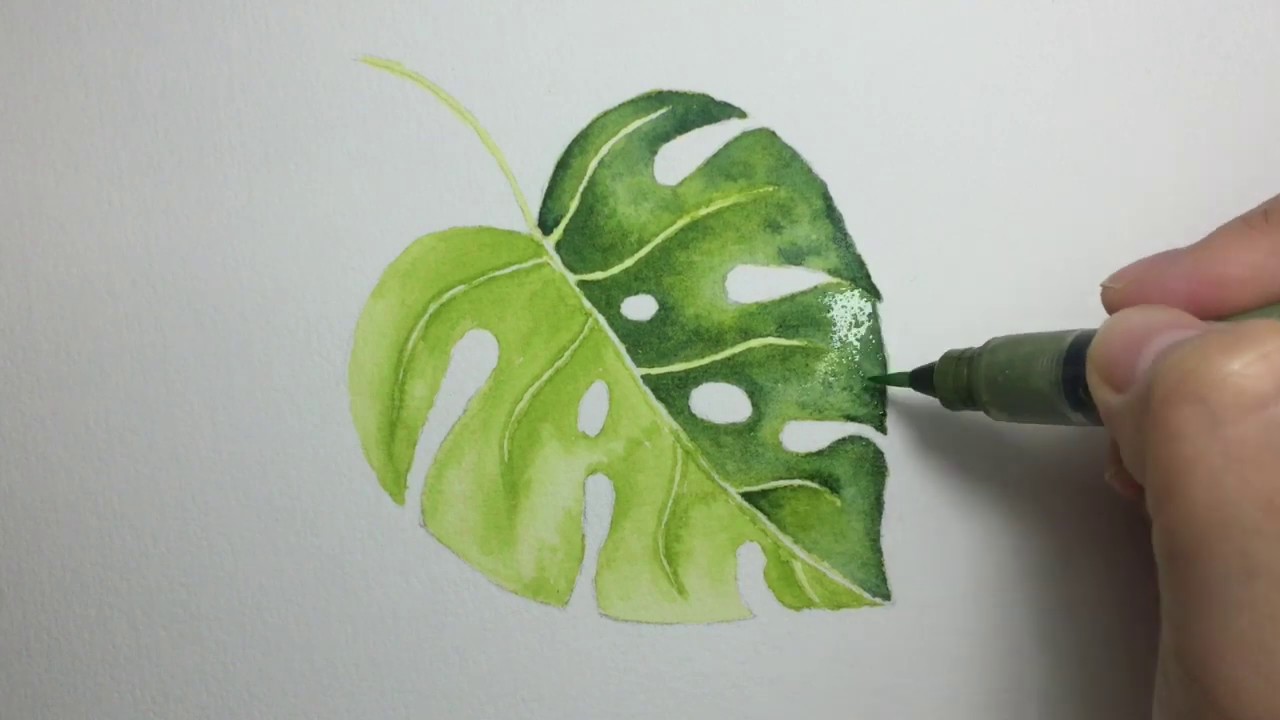The image, framed in a horizontally rectangular format without a border, depicts a detailed and vibrant scene that takes place indoors under artificial lighting. The background is a flat, gray tone that contrasts with a crisp white sheet of paper at the center. On this paper, an intricate leaf drawing is being crafted by an artist who holds a dark green marker with their thumb and forefinger—both part of a white hand visible on the right side of the image. The leaf features a stem and a heart-shaped structure with two distinct shades of green: the right side is darker while the left side is lighter. The texture of the leaf hints at a watercolor-like effect despite the use of a marker, and the ink appears so wet that it almost reflects the light. The leaf is meticulously detailed with several holes of varying shapes—some teardrop-shaped, others more oval—strategically placed both in the middle and along the edges of the leaf, enhancing the sense of artistic depth and precision.